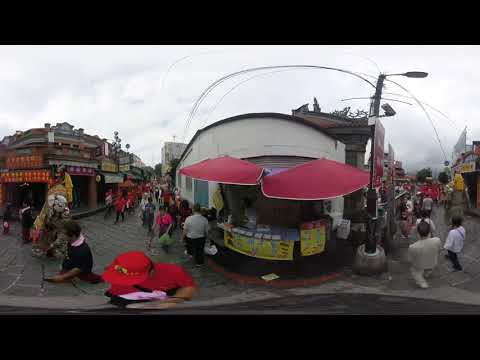The photograph captures a bustling outdoor market scene, likely set in an Asian country given the architectural details and cultural elements present. At the center, a prominent fixed food stand with bright red awnings draws attention, resembling a small building designed for selling goods or tickets. Dominating the scene is a man in a red hat and red shirt, serving as a focal point amid the crowd. The market is set against a backdrop of single-story buildings with garage doors indicating various shops inside, adorned with numerous shop signs extending into the distance. Cobblestone or brick-paved pathways weave through the market, populated by a diverse multitude of people, engaging in shopping or attending a festival-like event. The sky is overcast and gray, contributing to the scene's muted daytime ambiance. Additional features include a curved corner building at the center, extending to the left and right, and a noticeable street light adding to the urban setting. The overall panorama captures a dynamic and vibrant marketplace atmosphere.